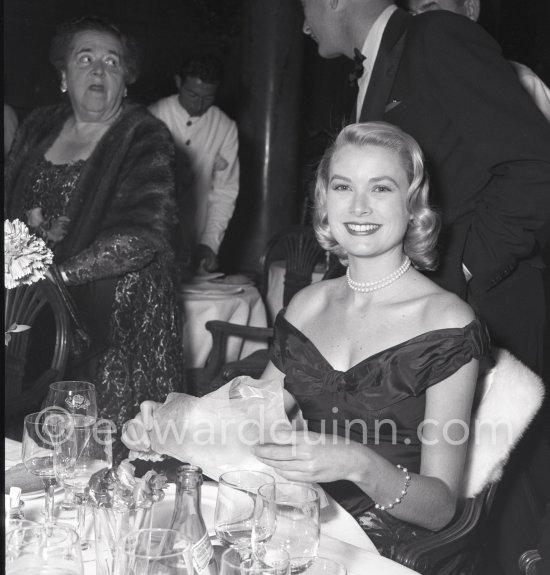This is a black and white, vintage photograph centered around a smiling woman seated slightly to the right of the frame. She has blonde, shoulder-length curly hair pulled back a bit, and is adorned in a black dress with a pearl necklace and a pearl bracelet on her left arm. In her hands, she holds a napkin or cloth. In front of her, a dining table displays several wine glasses and bottles, all set on a white tablecloth.

Behind the woman, a man in a suit or tuxedo, visible mostly from the left side, leans slightly as if speaking to another woman at a different table. This woman, located to the left, has shorter curly hair, is dressed in a black dress with a fur coat, and is engaged in the conversation with the man. In the farther background, there are additional tables covered with white tablecloths and a waiter dressed in a white suit looking down at one of the tables.

The photograph bears a watermark at the center bottom, which includes a copyright symbol and a partially legible domain name, resembling 'ewaydarkwin.com,' in a translucent font that blends with the monochrome aesthetic.